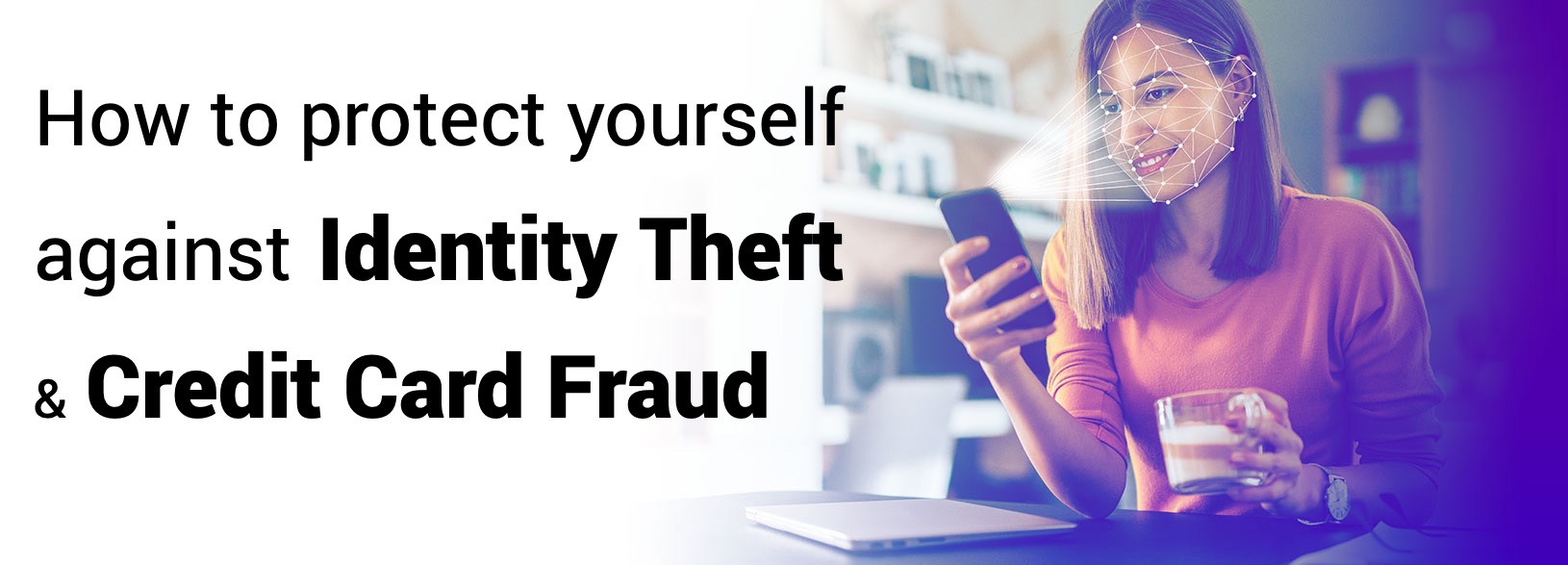This image, which appears to be an advertisement, is focused on the theme of identity theft and credit card fraud prevention. On the left side of the image, bold black text reads, "How to Protect Yourself Against Identity Theft and Credit Card Fraud," set against a white background. The right side of the image features what appears to be a stock photograph of a woman in her late 20s. She has just-below-shoulder-length brown hair and is seated at a desk in what looks like a home office, identifiable by the visible shelf and photographs in the background.

The woman is casually seated in front of a closed laptop, wearing a salmon-colored sweater and a smartwatch. She is holding a mug in her left hand and a smartphone in her right hand, which she is intently looking at. Above her face, beams of light emanate from the smartphone, converging on her facial features. Overlaid on her face are geometric patterns of connected triangles with dots, giving the impression that the phone is scanning or measuring her face. This visual effect underscores the message of the text, highlighting concerns about personal security in the context of digital identity verification.